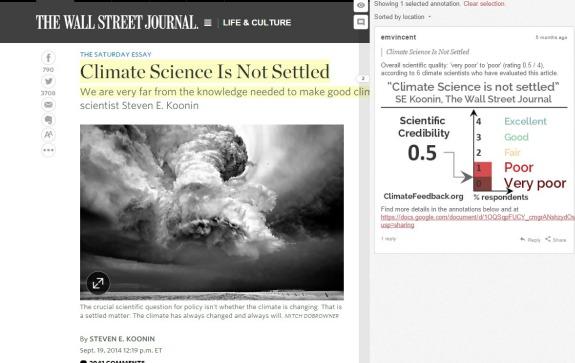The image features a black background with white text and various elements that appear to be part of a digital article layout, specifically from The Wall Street Journal. At the top, "The Wall Street Journal" is prominently displayed in bold white text. Next to this title are four small bars, followed by the label "Life & Culture."

In the top-left corner, there are two small squares. The first square is white with a gray eye icon, and the second square has a gray speech bubble icon. Running down the left side of the image are social media and interaction icons, including the Facebook logo with the number 790, the Twitter logo with the number 3702, followed by mail and several other unidentified icons, including an uppercase/lowercase 'A' and three dots.

On the right side, the text "The Saturday Essay" is in gray. Below this, in black text outlined in yellow, it reads "Climate Science Not Settled." The text continues with "We are far from the knowledge needed to make good," but it is cut off at "Clin." 

Underneath, in black text, the caption reads "Scientist Steven E. Kuhn." An image of black-and-white clouds follows, with illegible white text overlaid. Below the image, it states "by Steven E. Kuhn, September 19th, 2014, 12:39 PM ET."

Additionally, on the right-hand side, there is a gray box with black text that says, "Showing One Scheduled Antidote Clear Sections Sorted by Location," followed by "Sentences Something About Environment." The text "Climate Change Not Settled, Scientific Credibility is 0.5" appears, indicating a poor quality article. The overall design and textual content contribute to a cluttered and confusing appearance.